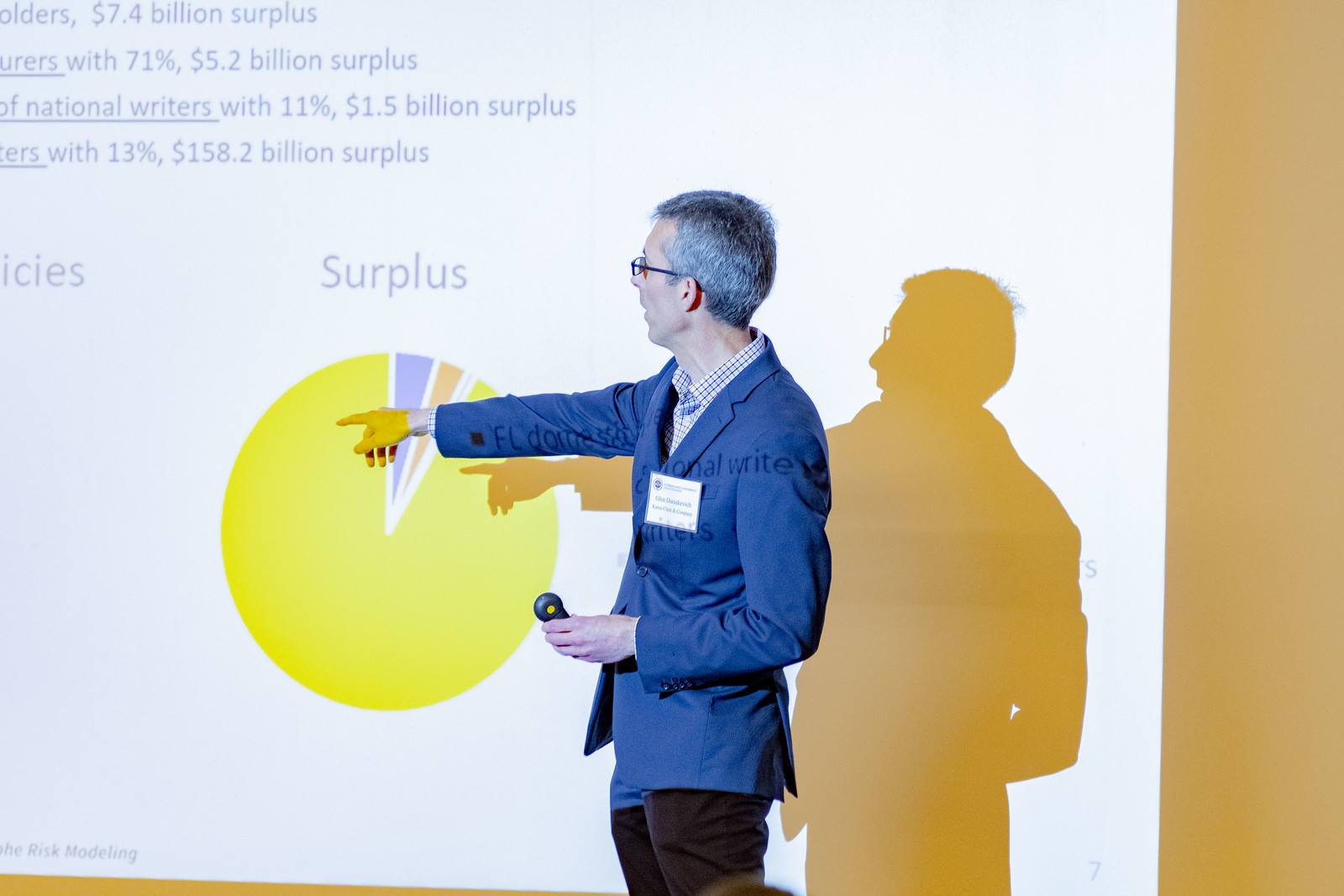The image is a wide rectangular color photograph of a man giving a presentation in front of a projected slideshow on an off-white, yellowish wall. Positioned in the center, the man has fair skin, short gray hair, and is wearing glasses. He is dressed in a blue suit jacket over a light blue plaid collared shirt, paired with dark trousers. A large white name tag is attached to his lapel. 

He is pointing to the left with one hand while holding a remote in the other. The projection behind him displays a yellow pie chart labeled "Surplus" with small purple and orange slices, and various text figures including, "Older's $7.4 billion surplus," "71% $5.2 billion surplus," "Of National Writers, 11%, $1.5 billion surplus," and "13%, $158.2 billion surplus."

His posed gesture casts a distinct shadow on the wall to his right, mirroring his stance. The man appears to be explaining the pie chart, which predominantly features yellow with small sections in other colors to illustrate specific data points.